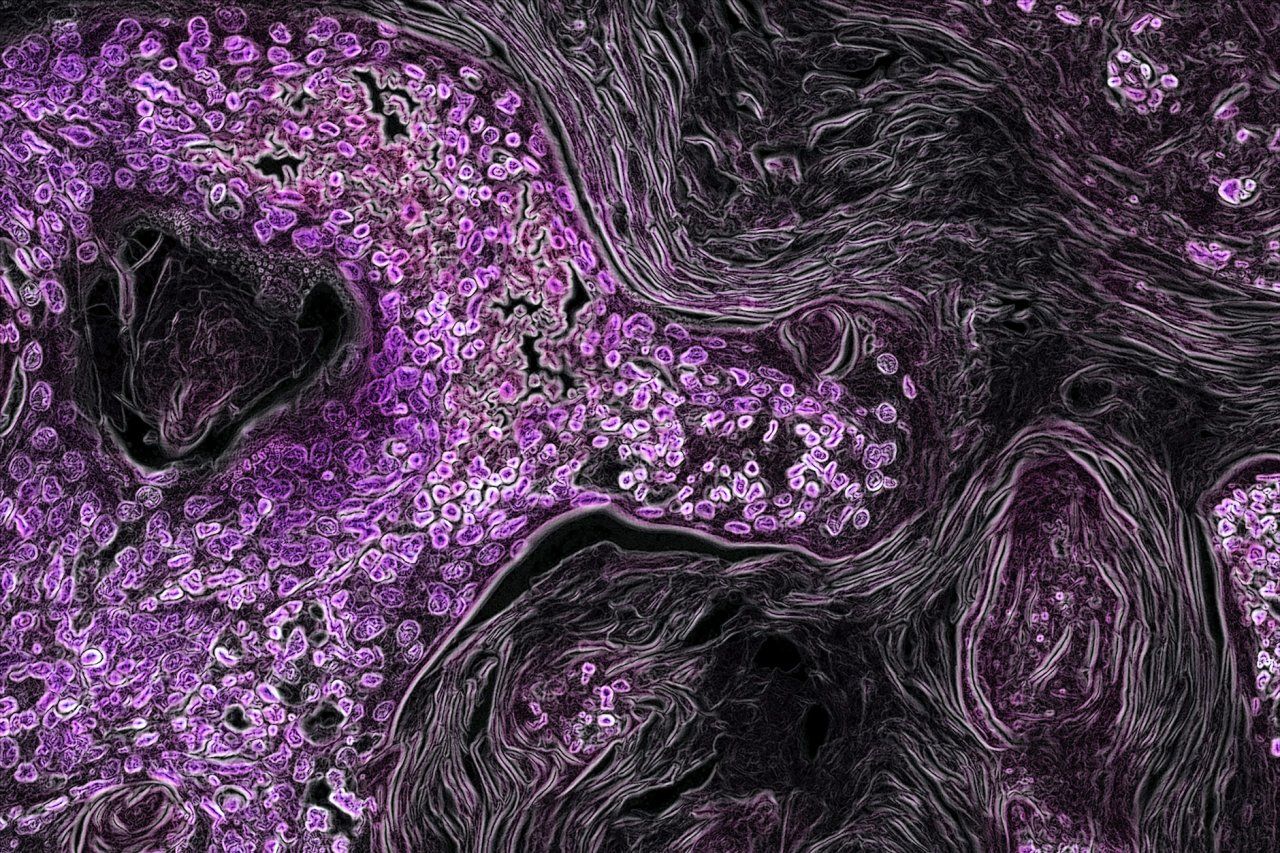The image appears to be an abstract or microscopic representation, likely digital artwork or a scientific visualization. It predominantly features black wavy and fibrous structures intertwined with small lavender and pink blobs resembling amoeba or cells. These cellular-like forms have dark purple or pink centers bordered by lighter shades of the same colors, creating a striking contrast. The left side of the image is particularly crowded with these lavender and pink round shapes, which seem to float around a larger black mass. Throughout the image, scattered black and grey streaks and dots add complexity, some forming small ovals and wavy patterns. There's a noticeable dark triangular section with black spots in the top left corner, and an overall purple tinge against the backdrop of a mix of greyish white. This enigmatic illustration could be a digital painting, a piece of abstract art, or a digitally enhanced microscopic image possibly colored for clarity in medical or scientific usage.